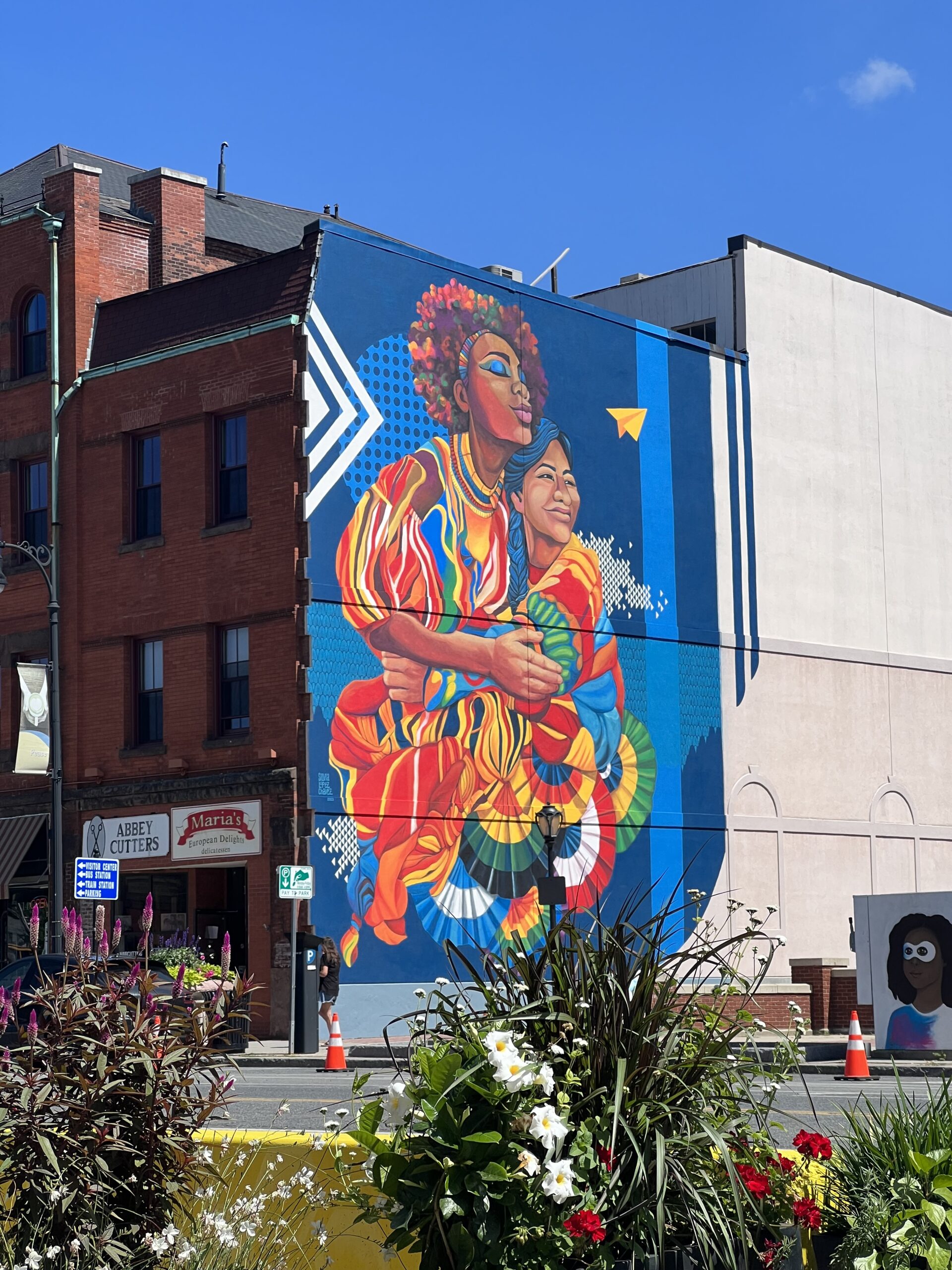The image features a daytime street scene centered on a tall brick building with a striking blue mural painted on its side. The mural, which covers the entire height of the building, depicts two women of diverse backgrounds—one Black and one Indian—embracing warmly. They are adorned in vibrant, colorful clothing with stripes and patterns in reds, blues, greens, yellows, and oranges. Above them, a yellow paper airplane is streaking upward, adding a whimsical touch. The background of the mural is primarily blue, accentuated with white triangular designs.

On the front of the brick building, above a glass door or window, a white sign reads "Abbey Cutters." Adjacent to this is a rectangular white banner with red text that says "Maria's European Delights." The building itself is situated across from a park with tall grasses and an array of red and white flowers, which appear in the bottom of the frame. Safety cones are positioned on the sidewalk next to the building, adding to the urban ambiance. The image captures a clear blue sky, emphasizing the bright and lively atmosphere of the scene.